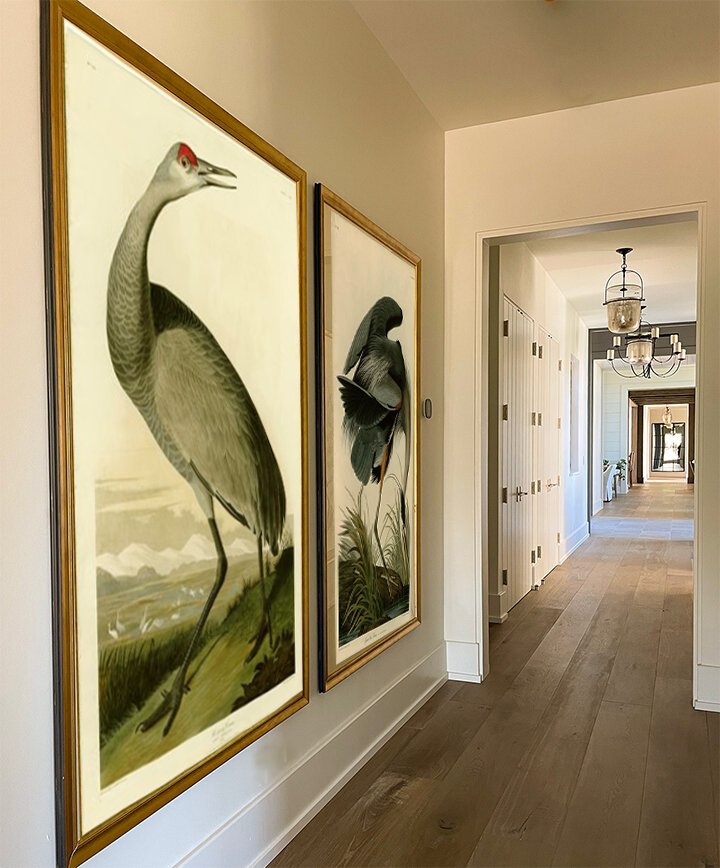This photograph features a long, narrow indoor hallway with wooden, beige-ish floors and cream-colored walls. The left wall is adorned with two large, gold-framed paintings, each around 6 feet tall, depicting birds. One painting features a white crane with a red head standing on grass, while the other shows a bird with a greenish-gray and black coloration, its neck angled downwards towards the water. Further down the hallway, beyond the paintings, there are two white closet doors. Overhead, several white chandeliers and lights hang from the ceiling. The corridor appears to be part of a large mansion or estate, stretching extensively in length and capturing a sense of grandeur.